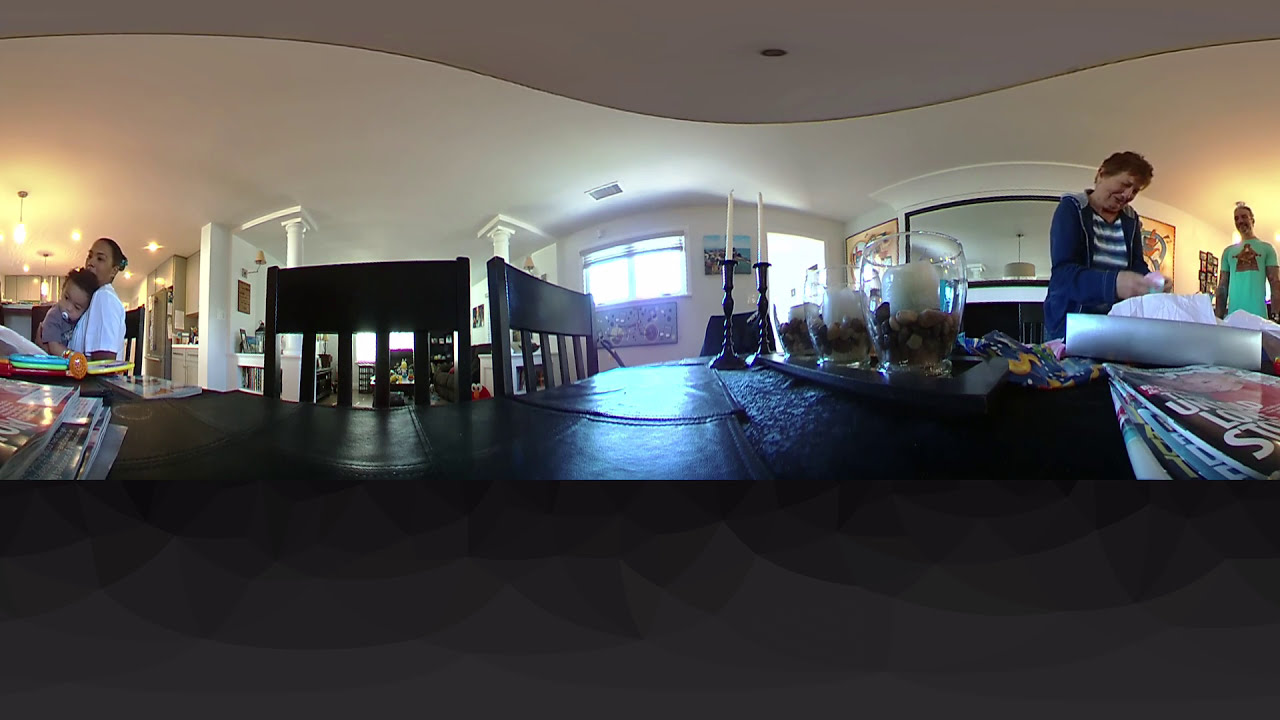The image, taken with a fisheye lens, offers a wide-angle view of a family preparing for dinner in a bright, white-walled room. The room features white ceilings, some white pillars on the left, and a large window and door in the center leading to another room. There's a large mirror with paintings hanging on either side on the far wall. In the center of the scene is a dark wooden dining table cluttered with magazines, tissue boxes, baby toys, and two white wax candles.

On the left side of the table, a brown-skinned woman is holding a small child with a pacifier in its mouth, likely trying to keep the child entertained. Toys are scattered in front of them, and a stack of magazines sits nearby. The woman appears to be wearing a zip-up sweater, suggesting she is in a relaxed and casual home setting.

On the right side of the table, an older woman with short hair, wearing a blue hoodie over a blue and white striped shirt, is seen peeling vegetables into a plastic bag. She might also be opening gifts, as there is pink packaging and she holds something pink in her hands. Behind her, a man in a mint green t-shirt stands observing and smiling, possibly her son. The chairs around the table are tall and wooden, adding to the cozy, homey atmosphere of this family gathering.